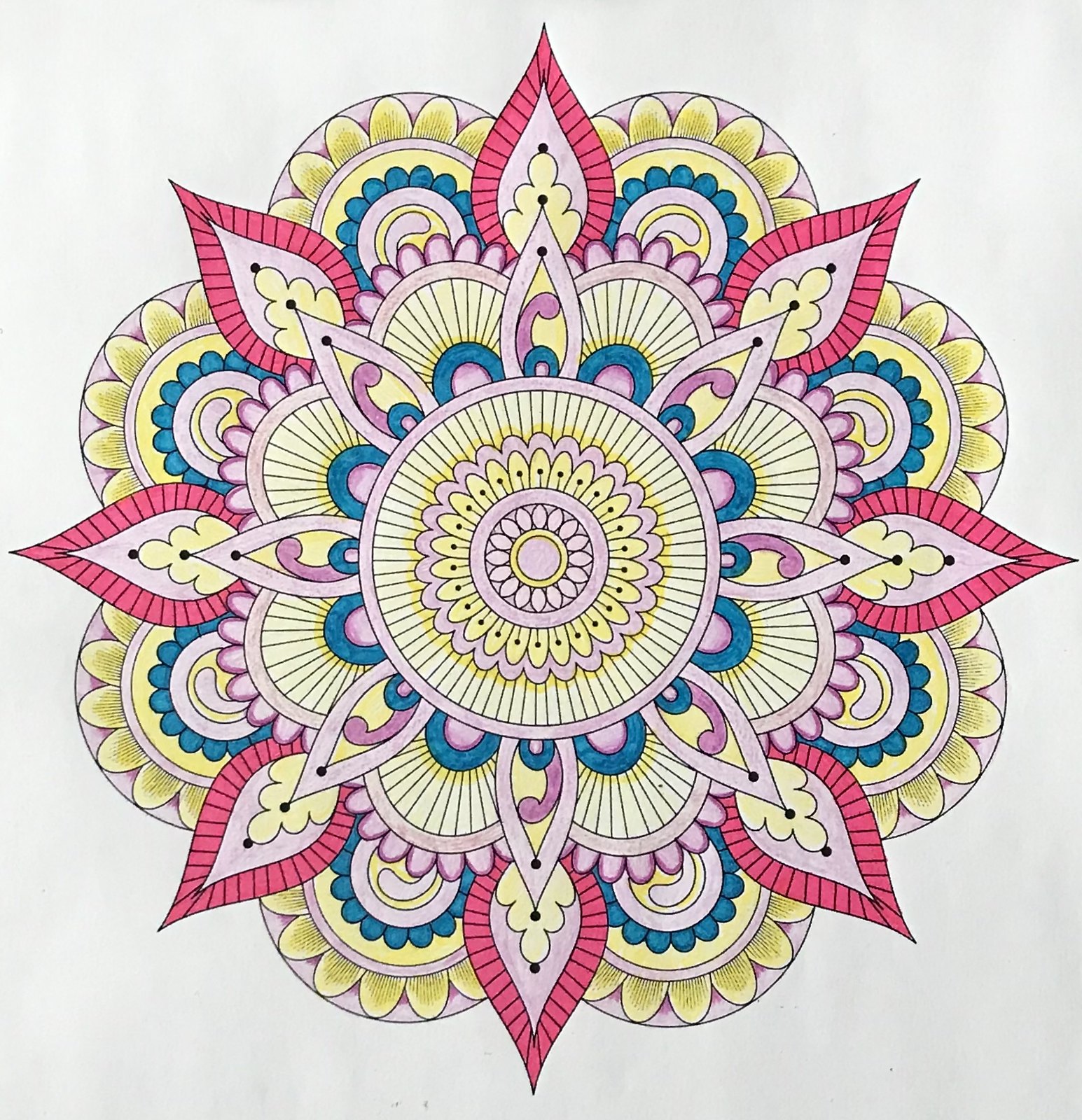This image showcases a meticulously detailed, computer-generated geometric drawing, reminiscent of designs typically found in coloring books. The composition primarily features an intricate floral pattern, with various layers and colors contributing to its complexity. At the base, the flowers display broad, rounded petals painted in vibrant yellow, each with smaller blue petals nestled within them. The interplay of yellow, blue, and occasional white spaces adds depth to this section. Moving upwards, the floral layers become more diverse and colorful. Midway, the flowers take on a combination of purples and pinks, creating a visually appealing transition. At the top, the flowers become distinctly pointy, predominantly pink with black accents, adding a bold contrast to the softer hues below. The overall effect is a mesmerizing blend of geometric precision and artistic creativity.